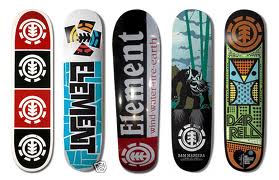This is a photograph of five snowboard decks standing on end against a white background. Each snowboard features a unique design. The deck on the far left has a white border and is divided into four alternating red and black squares, each containing a circular symbol with a plant-like emblem inside. To its right, the second deck has a two-tone white and blue design with the word "element" in black letters on the blue portion. The third snowboard from the left is primarily black and red, divided into separate halves with the word "element" in white on the red bottom half, and featuring the same circular plant emblem. Next, the fourth deck has a blue background resembling gray rocks underneath and showcases the white circular plant emblem prominently. On the far right, the fifth snowboard is decorated with a red circle at the top over a green, blue, and red patterned background, and includes a cubic depiction of a bird.